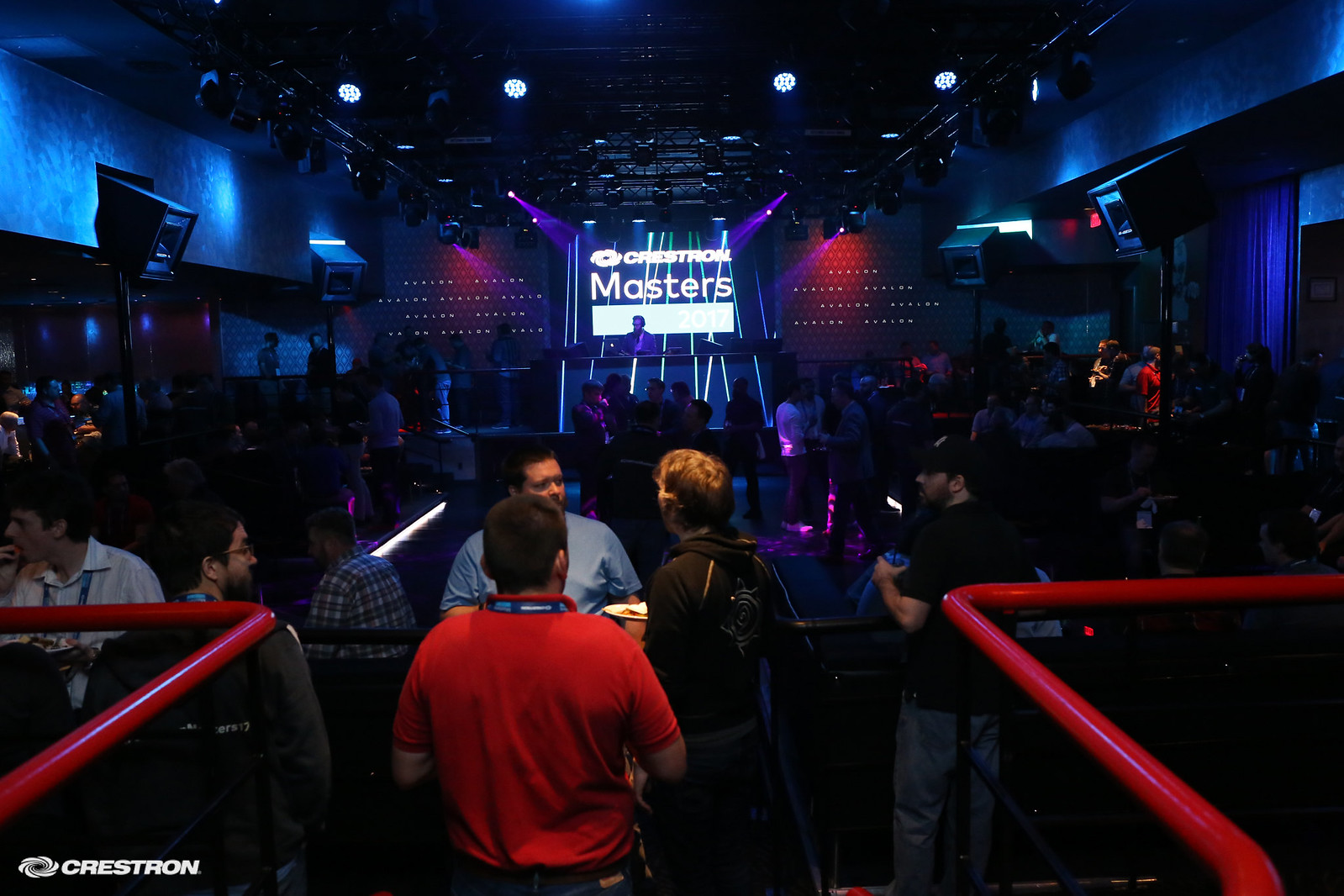The image depicts a lively indoor scene that appears to be set in a dimly lit nightclub or party venue. In the foreground, two red bars are visible in both the bottom left and bottom right corners. At the center of the photo stands a man in a red shirt, wearing a name tag or lanyard around his neck, visible from the back. Surrounding him is a crowd of people, predominantly men, engaging in conversation and holding drinks. To the left, a man in a white shirt, also wearing a lanyard, is seen eating. Another individual in front of the man in red is wearing a black jacket and holding a plate.

In the background, a DJ is positioned at a booth, illuminated by purplish lighting. Above him, large speakers protrude from the walls. A screen or projection behind the DJ displays the phrase "Crystal Masters" or "Crest Ron Masters," while the words "Avalon" are repeatedly visible on either side of the DJ booth. The setting exudes an atmosphere of a music party or some kind of informal gathering, with people mingling and enjoying themselves amidst the dim lights and energetic ambiance.